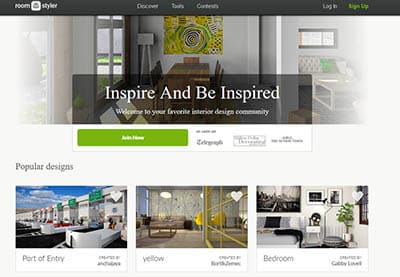In this image, set against a pristine white background, is a small yet detailed screenshot of a webpage. While the company name isn't legible, the text in the upper left corner appears to partially read "room." In the upper right corner, there are slightly blurred words indicating a "log in" option, with another indistinct phrase in green text next to it. Dominating the center of the screenshot is a vibrant color photograph showcasing a beautifully designed modern living space. The room features immaculate white walls adorned with a striking large canvas painting. There's a long, minimalist brown wooden table flanked by chairs on both the right and left sides. On the far right, the image hints at a blurred vision of a white couch paired with a sleek white cocktail table. Bold white text overlaying the image reads, "Inspire and be inspired. Welcome to your favorite interior design community."